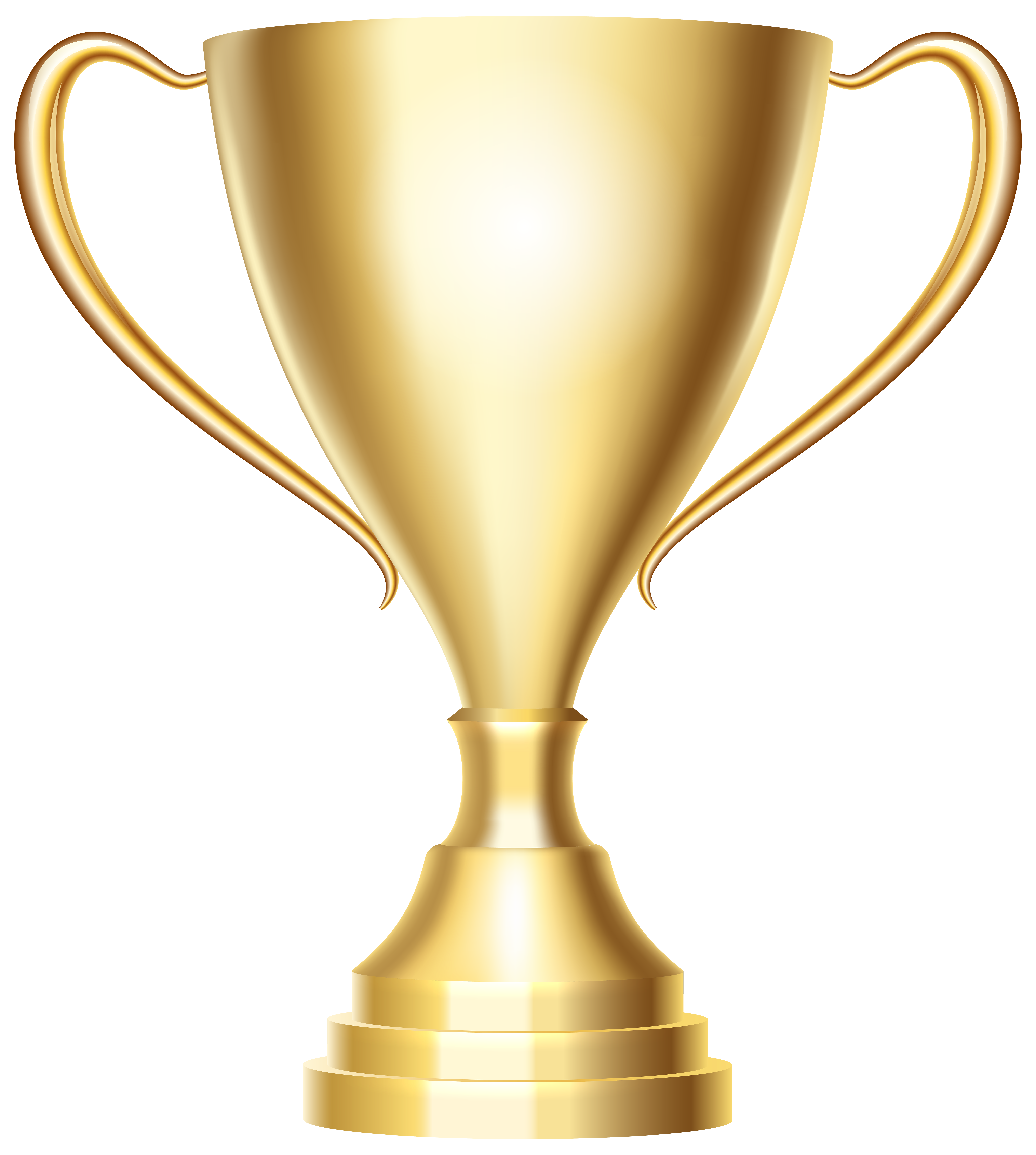The image features a digitally rendered, shiny gold trophy set against a stark white background, so white that the edges blend into the surroundings, making it difficult to discern where the trophy begins and ends. The trophy resembles a large goblet with two handles, one on each side, forming almost a heart shape, suggesting it could be grasped and lifted as if to drink from it. The design is simple yet elegant, with a base composed of three descending tiers leading to the narrower stem that supports the wide cup at the top. There are no inscriptions or designations indicating a specific award or competition. Shadows are visible on either side of the trophy, emphasizing its shiny and reflective gold surface. The overall appearance is more of a stereotypical, computer-generated golden trophy rather than a highly detailed, realistic one.